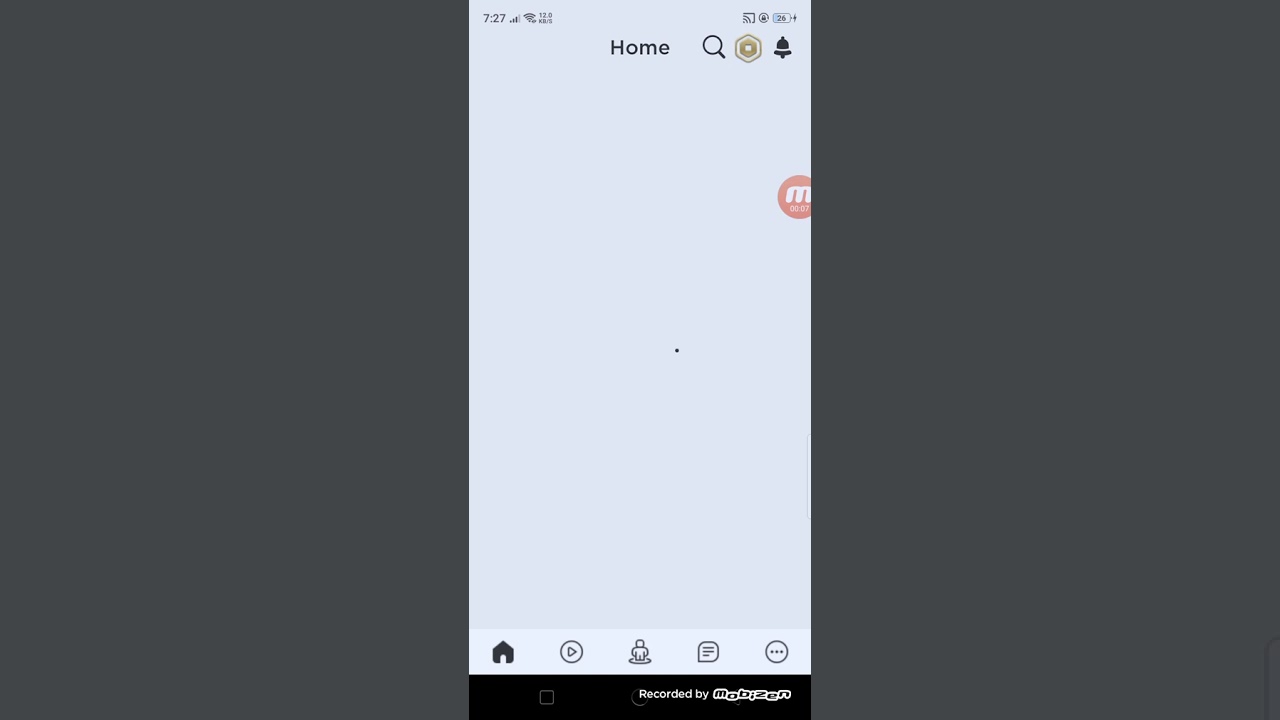The image displays a screenshot of a phone screen with a distinctive aspect ratio, being approximately 50% wider than it is tall. The image is heavily letterboxed on both sides, with about 35% of the width on the left and right sides covered by a very dark gray border, as opposed to the usual black letterboxing. 

At the center of the image, the background features a light blue-gray hue. In the upper left corner of the screen, black text reads "727," accompanied by a signal icon. Moving to the upper right, there are several additional icons, including a battery meter indicating roughly two-thirds charge.

Prominently in the center of the screen, the word "Home" is displayed in large black font. To its right is a magnifying glass icon, followed by a few more icons. The majority of the screen is blank, except for an "M" that seems to float within a circle. This circle is positioned about a third of the way down on the right side of the screen and is cut off approximately 20% from the right edge. The circle housing the "M" is light red, creating a striking visual that suggests the icon is slightly offset to the right.